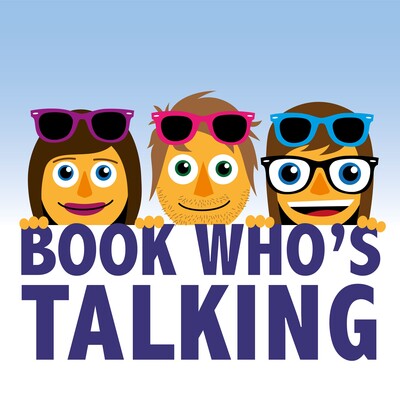The image is a cartoon poster featuring three illustrated faces in a row, each peering up and appearing to have their hands on the edge of a text block. The background is divided into two shades of blue, with a lighter blue behind the faces and a darker blue behind the text. 

On the left is a smiling woman with long brown hair and blue eyes, adorned with purple sunglasses sitting on her forehead and wearing purple lipstick. In the middle is a man with light brown hair, a rough stubbly beard, and green eyes, with pink sunglasses perched on his head. On the right is a grinning woman with brown hair and blue eyes, sporting regular eyeglasses with a black frame and blue sunglasses on her forehead. Beneath the three faces, against a white background, the text in purple reads, "Who's Talking?"